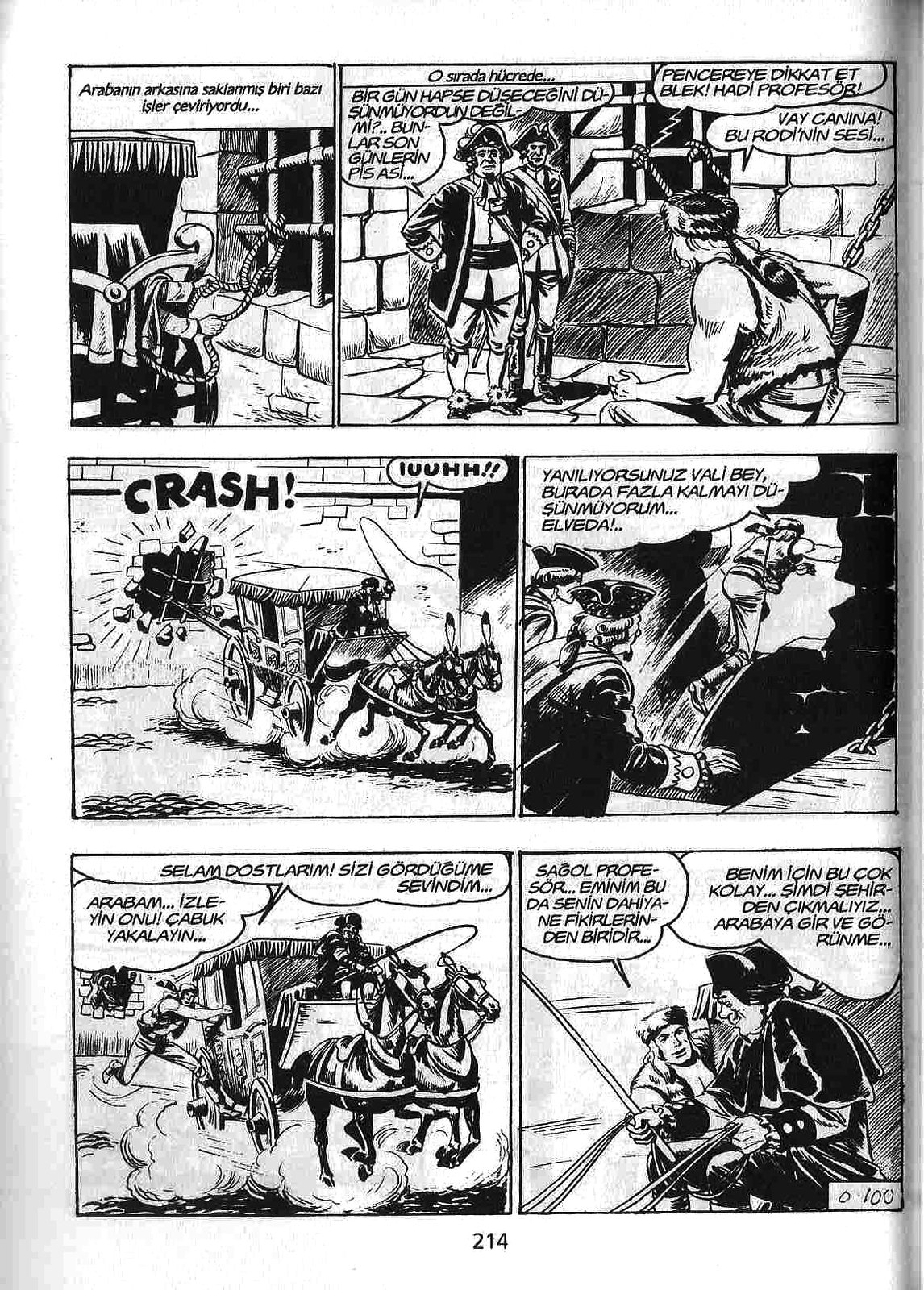This vibrant comic book page, likely from an action-packed historical or adventure series, is composed of six vividly detailed panels, each rich with colorful illustrations and foreign-language dialogue, possibly Eastern or Western European and including phrases that suggest a blend of Germanic and Romance languages. 

The first panel features a stationary stagecoach, set in a period scene with intricate details. Text bubbles in the panel describe the scene in a foreign language, with phrases like "Arabian Arkansas" and other decipherable words suggestive of place and context. 

In the second panel, colonial-era soldiers, dressed in 18th-century uniforms, are seen interacting with a man wearing a Davy Crockett-style coonskin cap. The scene depicts the man in the coonskin cap seated in a jail cell, conversing with what appears to be a captain and another officer standing outside the cell door, their words peppered with phrases like "Pen serrati docot."

Moving to the third panel, the chaotic scene shows a stagecoach, now pulled by horses, dramatically crashing through a wall or barrier. The sounds and exclamations are captured in expressive lettering, complementing the action-packed visual. 

The fourth panel continues the story as the men in revolutionary attire, including the Davy Crockett figure, use the breach in the wall to make their escape. The text here, again foreign, conveys urgency and spirited commands.

In the fifth panel, the illustration captures the man in the coonskin cap as he leaps onto the stagecoach, the text describing this daring move. 

Finally, the sixth panel focuses on the stagecoach driver, who is in the midst of a tense moment, with someone attempting to jump into the moving vehicle. Dialogue continues in the foreign language, adding an element of mystery and excitement to the scene. This panel concludes the page with the words "Salaam post Lam" and other fragmented phrases.

Overall, the page is a dynamic blend of action and dialogue, richly illustrated to transport the reader to an adventurous historical setting, with the final panel hinting at further suspenseful developments.